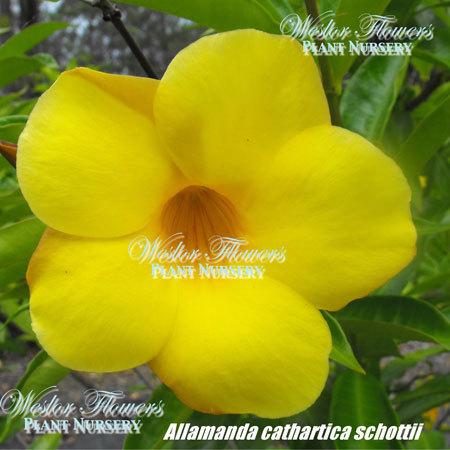This outdoor photograph showcases a close-up of a large yellow Allamanda cathartica schottii flower at the center, surrounded by a backdrop of blurred green leaves. The flower, composed of five spacious petals tinted with slight orange accents at their edges, features a deep, brownish-orange center. Superimposed across the image, the brand name "Wester Flowers Plant Nursery" appears multiple times—clearly visible in the central area, upper right-hand corner, and lower left-hand corner, although the overlapping logos create a blurry appearance in some spots. The plant's scientific name, "Allamanda cathartica schottii," is written at the bottom of the image. This scene captures a bright, midday garden setting.